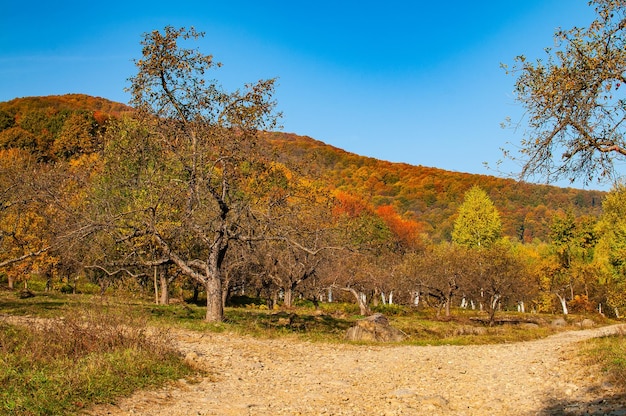The image depicts an autumnal setting in the foothills of the mountains, showcasing a brilliant, cloudless blue sky. The mountains in the background are densely covered with trees in varying stages of foliage change, exhibiting a mix of green, red, orange, and brown hues. In the mid-foreground, there is a prominent large tree, which has branches sprawling in every direction; its leaves are mostly green but starting to exhibit signs of seasonal change, with some top branches baring sparse leaves, as though autumn has begun its work. A gravel path enters the scene from the front and bifurcates midway into the image, leading into a fork nestled with a cluster of trees resembling a pruned orchard. The trunks of these shorter trees appear wrapped with tape, giving them the appearance of fruit trees. Beneath the trees, patches of grass add texture to the scene, completing this serene autumn landscape.